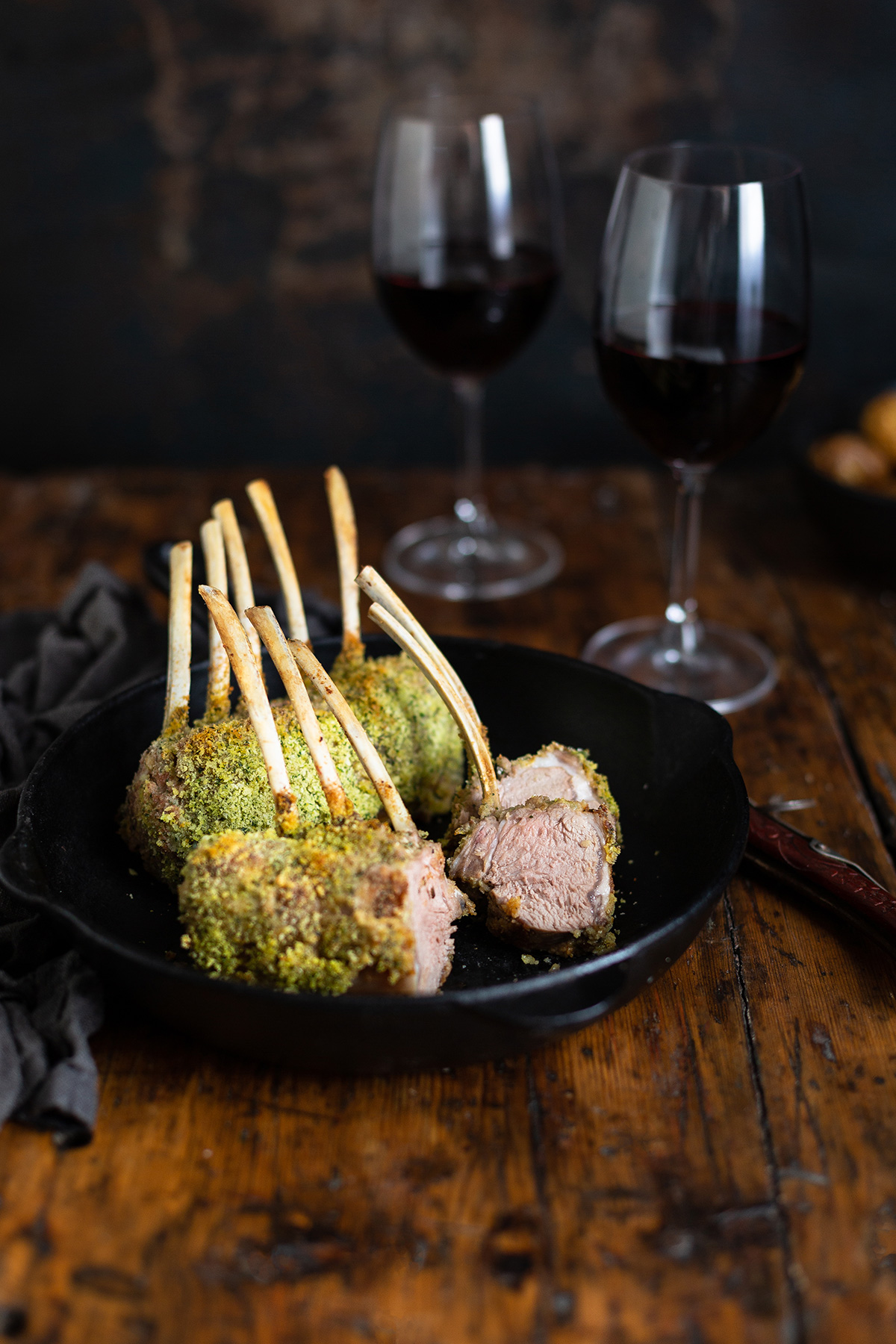The image captures a rustic yet elegant dining setting centered around a beautifully prepared rack of lamb. The lamb, encrusted with a vivid green pistachio and herb crust, is arranged in a black cast iron skillet, likely the same vessel used for searing and finishing the meat in the oven. The bones of the lamb stand upright, adding to the dish’s visual appeal, with one piece sliced to reveal the tender, juicy, pinkish center. This striking presentation rests on a dark, weathered wood table adorned with character-revealing scratches and knots. To the left of the pan lies a dark gray napkin, while on the right, partially tucked under the skillet, is a red-handled utensil. In the background, two elegant wine goblets filled with rich red wine hint at the meal’s sophistication. Faintly visible are additional dining elements, such as what appears to be bread rolls, enhancing the overall ambiance of a professionally lit photograph that could easily grace the pages of a gourmet food blog.